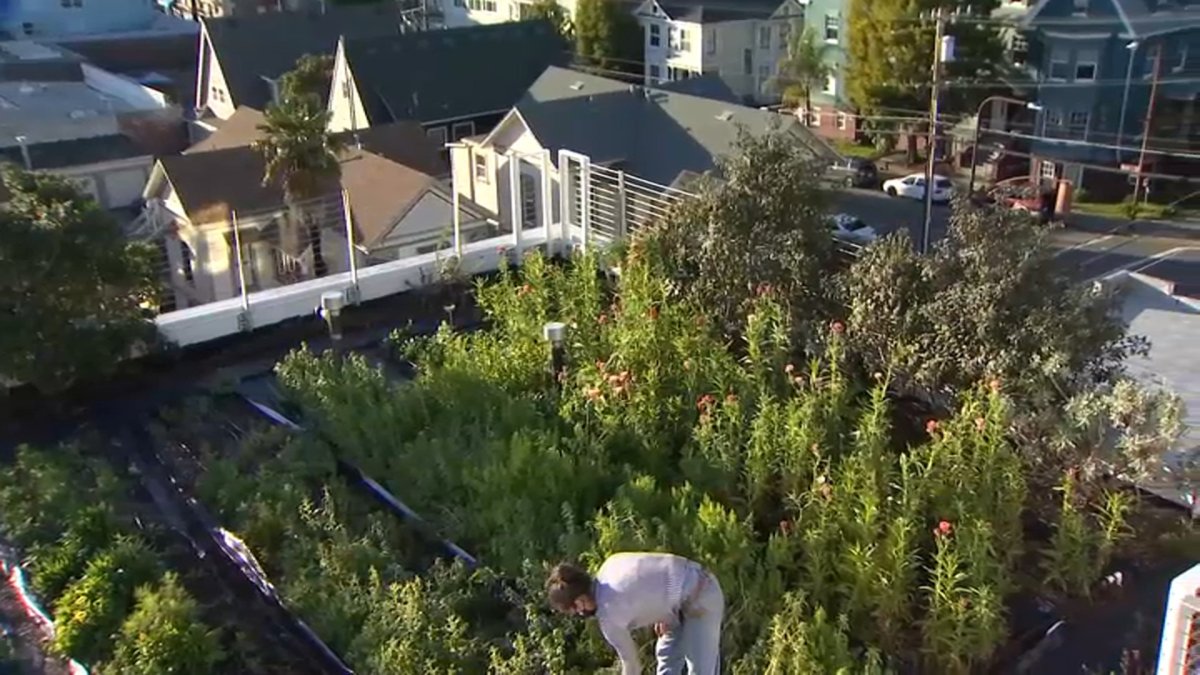This horizontal image captures an aerial view of a vibrant rooftop garden. Dominating the foreground is a woman, seemingly engaged in caring for the plants, her posture bent forward as she tends to the lush greenery. The garden itself features organized rows of various vibrant green plants, separated by strips of black plastic—indicative of thoughtful cultivation. 

On the periphery, particularly in the back left and right corners, stand smaller trees, possibly fruit-bearing, adding vertical interest to the garden's design. Beyond the immediate rooftop, the image transitions into an urban landscape characterized by the grey, brown, and white hues of various rooftops and building tops, creating a stark contrast to the vivid greenery of the garden. In the right-hand corner, a street intersection is visible, adding an element of dynamic city life to the scene. This detailed juxtaposition between lush foliage and the structured urban environment highlights the harmonious coexistence of nature and urbanity in a city's skyline.